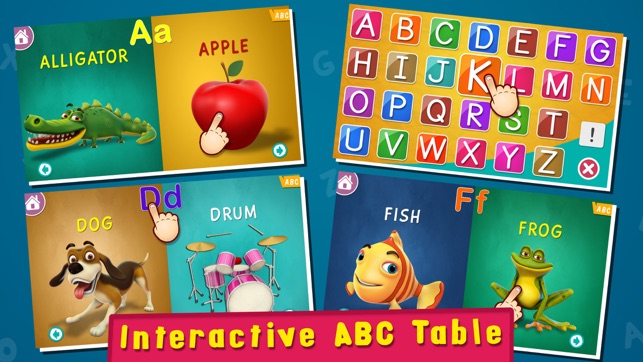This image features an interactive ABC table designed for children, showcasing whimsical and playful illustrations associated with each letter of the alphabet. The table includes endearing images like an alligator, apple, dog, drum, fish, and frog, each depicted in a charmingly absurd style. The dog, for instance, has a particularly comical expression with its tongue playfully sticking out. The drum is amusingly rendered with floating drumsticks, as if magically suspended in mid-air. Additionally, four pointing fingers are prominently featured, directing attention towards specific letters and their corresponding images: apple (A), drum (D), frog (F), and a fourth unidentified object corresponding to the letter K. Overall, the image captures a delightful and imaginative approach to early childhood education.